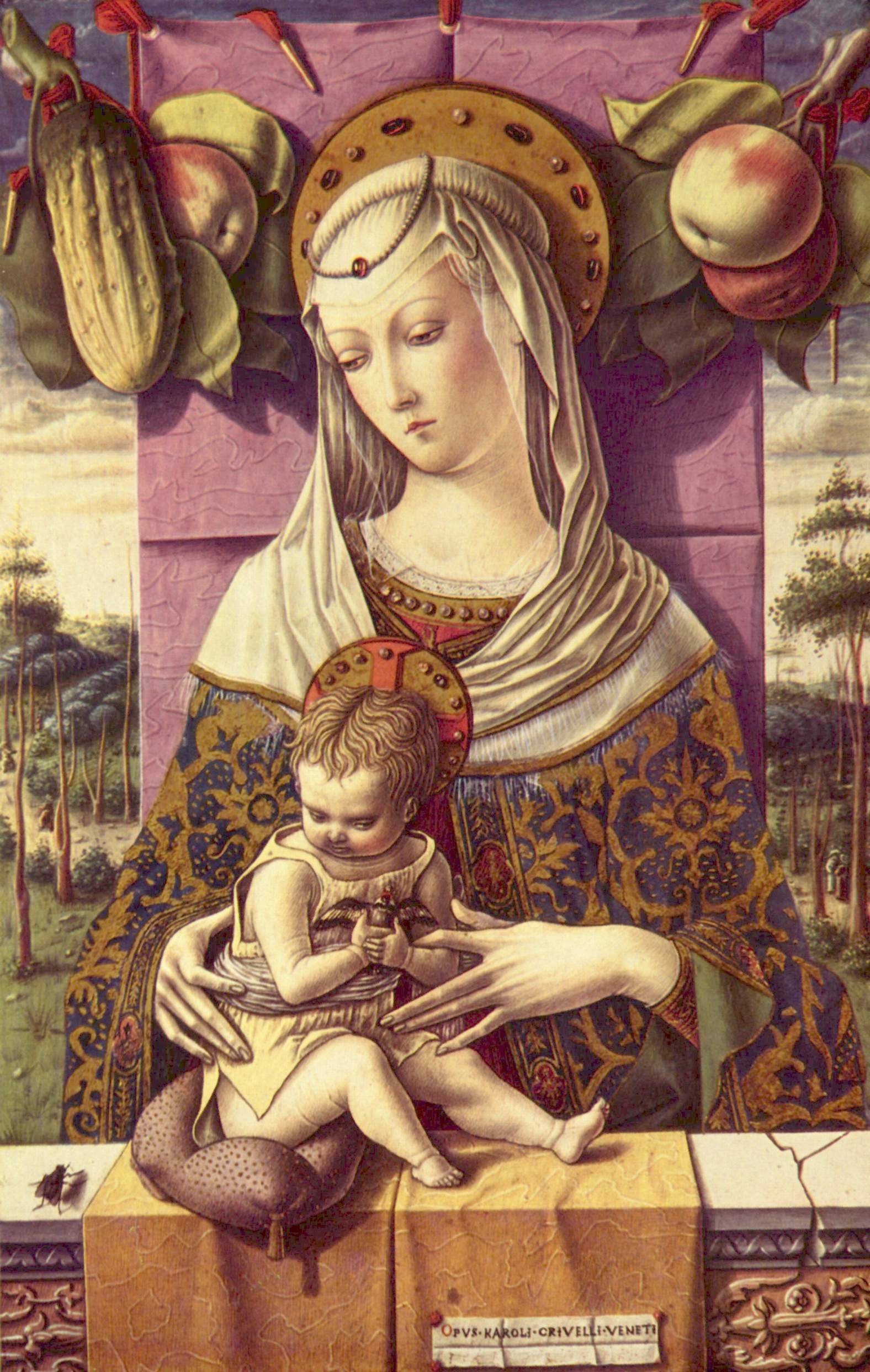The image is a detailed drawing portraying a woman, possibly Mary, and her child, likely baby Jesus, in a serene, contemplative scene. The woman, pale and appearing to be no older than her 30s, gazes downward to her right with a somber expression. She wears an ornate blue gown with gold accents and a white headdress adorned with a jewel headband on top. 

An angelic halo floats above her head, adding a divine aura to her presence. She gently holds the baby, who is dressed in a gown and seated on a cushion placed on a blanket that rests on a wall or fence. A white sticker or label can be seen affixed to the blanket. 

Above the woman's head, fruits like apples and vegetables like pickles or cucumbers are hanging, contrasting with the outdoor background that features several trees, a pathway, and distant hills. The purple or violet backdrop frames the scene, enhancing the spiritual and artistic quality of the drawing. A small fly can also be noticed on the wall in the lower left of the image, adding an intriguing touch of realism.